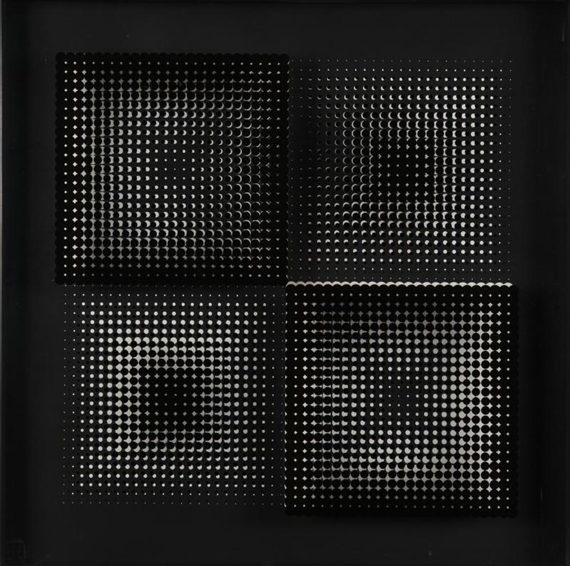The image is a large, solid black background featuring a centered arrangement of four squares, each composed of intricate black and white dot patterns creating optical illusions. The upper left-hand square has a darker black outline with a gradation fading into a lighter center dotted with tiny white and dark black spots. Adjacent to it, the upper right-hand square lacks a dark outline and focuses on a central dark background with half-moon shapes on the periphery. The lower left-hand square, without a prominent border, showcases mostly white spots with a dark central area, forming a star-like pattern extending outwards. The lower right-hand square, defined by a thicker black outline, appears lighter in the center. Together, these four squares crafted from smaller geometric shapes and dots create a mesmerizing black-and-white abstract artwork that challenges the viewer’s perception.